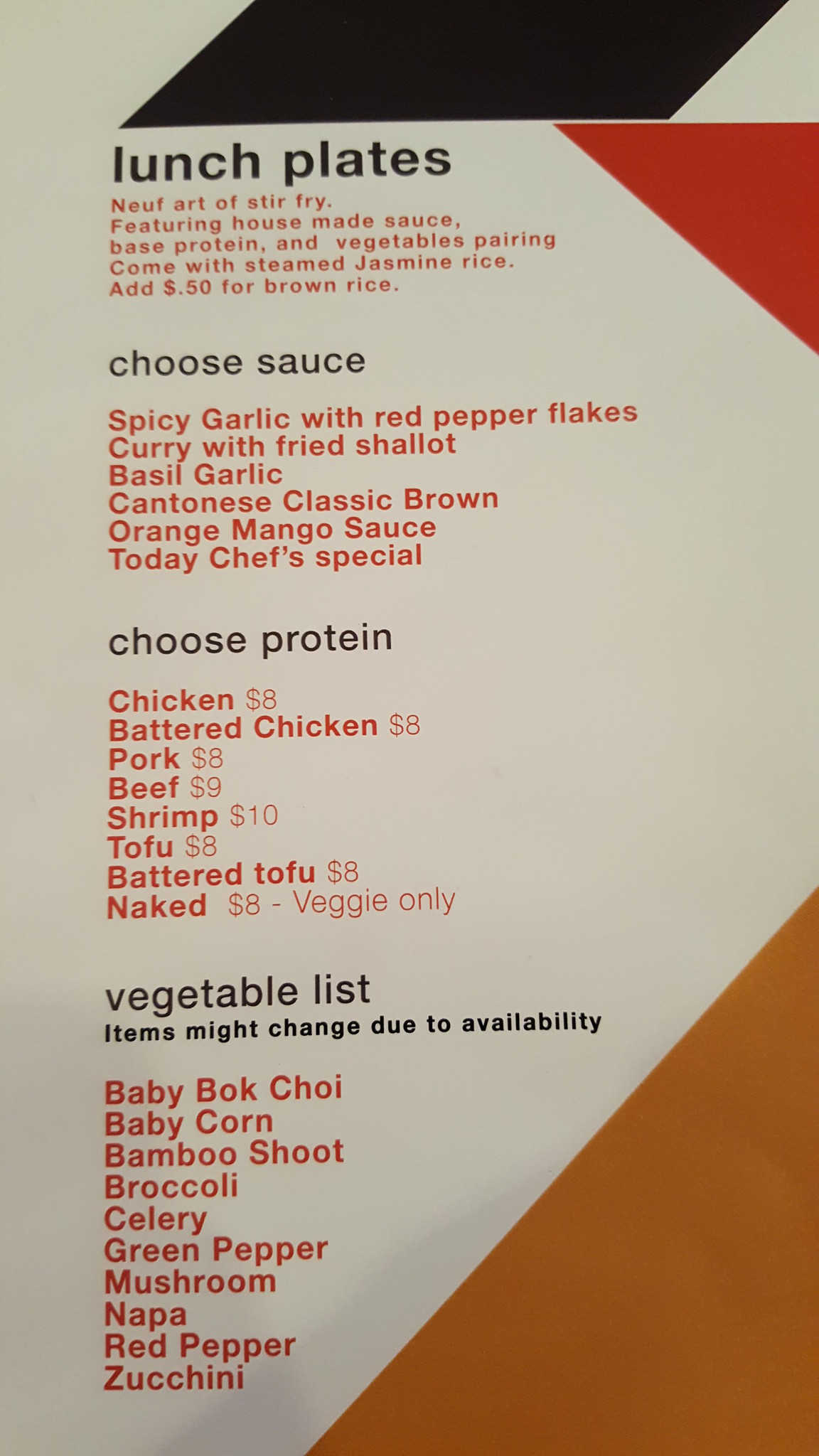**Menu Description: Modern Art Design**

The menu features a bold, modern art design on a white background. Across the bottom right corner, a large tan triangle extends from more than halfway across the bottom of the page to about a third of the way up the right side. Complementing the tan triangle, a smaller red triangle is positioned in the top right corner. Additionally, a black parallelogram is placed at the top of the page, creating a striking color-block composition.

The menu content itself is presented in a clean, simple font reminiscent of Arial. Each section header is in lowercase black lettering. Below the header, the text shifts to a rusty red-orange color.

**Sections:**

- **lunch plates:** 
  - *NEUF Art of Stir Fry featuring house-made sauce, base protein, and vegetable pairing. Comes with steamed jasmine rice (add $0.50 for brown rice).*
- **choose sauce:**
  - black text: *spicy garlic with red pepper flakes, curry with fried shallots, basil garlic, Cantonese classic brown, orange mango sauce, today's chef special.*
- **choose protein:**
  - black text: *chicken $8, battered chicken $8, pork $8, beef $9, shrimp $10, tofu $8, battered tofu $8, naked $8*
  - black text (separate line): *veggie only*
- **vegetable list:**
  - black text (note): *Items might change due to availability.*
  - red-orange list: *baby bok choy, baby corn, bamboo shoot, broccoli, celery, green pepper, mushroom, napa, red pepper, zucchini.*

This description effectively captures the essence of the menu's design and details the available dish options for a clean, modern dining experience.